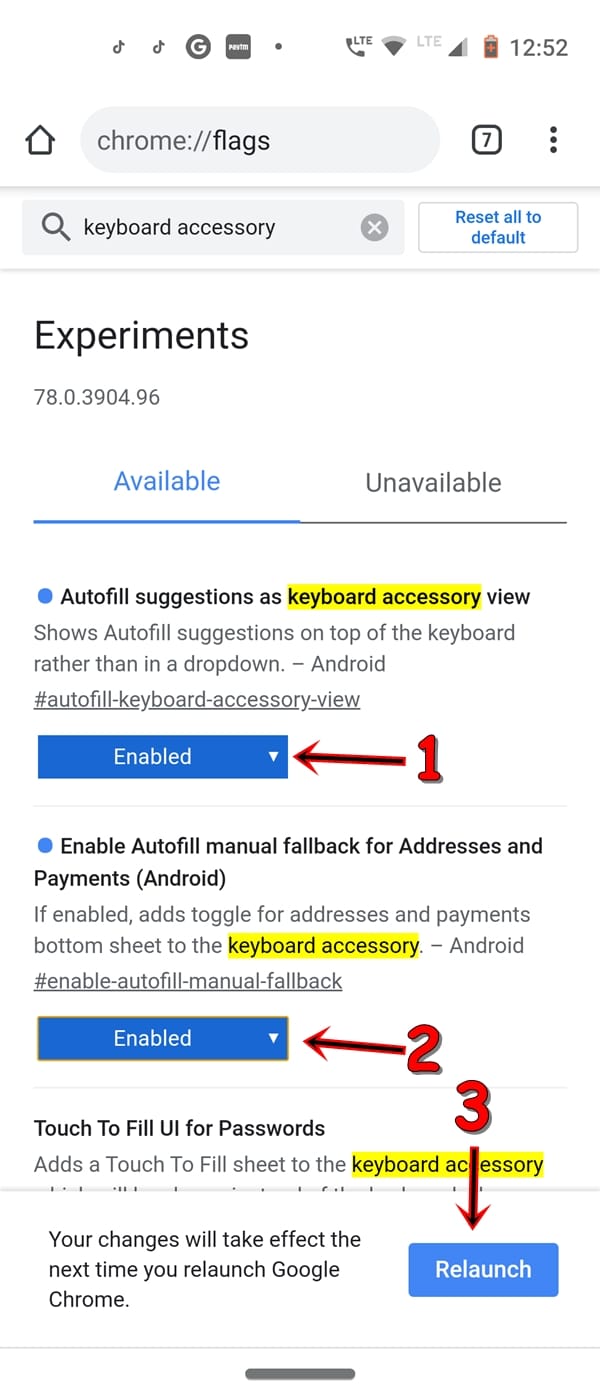A screenshot of a Chrome mobile browser displaying the 'chrome://flags' settings page. At the top, the URL is visible, followed by a search box with the term "keyboard accessory" entered. To the right of the search box is an 'X' button for clearing the search, and further right, a blue 'Reset all to default' option. The section cap reads 'Experiments' in bold black font, with the browser version number listed below. The page is divided into two sections: 'Available' and 'Unavailable,' with 'Available' underlined and highlighted in blue.

Vertically listed settings start with 'Autofill suggestions as keyboard accessory view,' where the term 'keyboard accessory' is highlighted in yellow. The description below this setting explains it, and a dropdown box to the right is set to 'enabled.' A hand-edited label marked '1' with an arrow points to this dropdown box. 

The second setting describes enabling autofill manual fallback for addresses and payments, specified for 'Android,' with the phrase 'keyboard accessory' again highlighted. This setting is also marked as 'enabled,' accompanied by another hand-edited label '2' with an arrow pointing toward it.

Towards the bottom right of the screenshot, a hand-edited label '3' points to a prominent blue 'Relaunch' button, signaling that changes must be restarted to take effect.